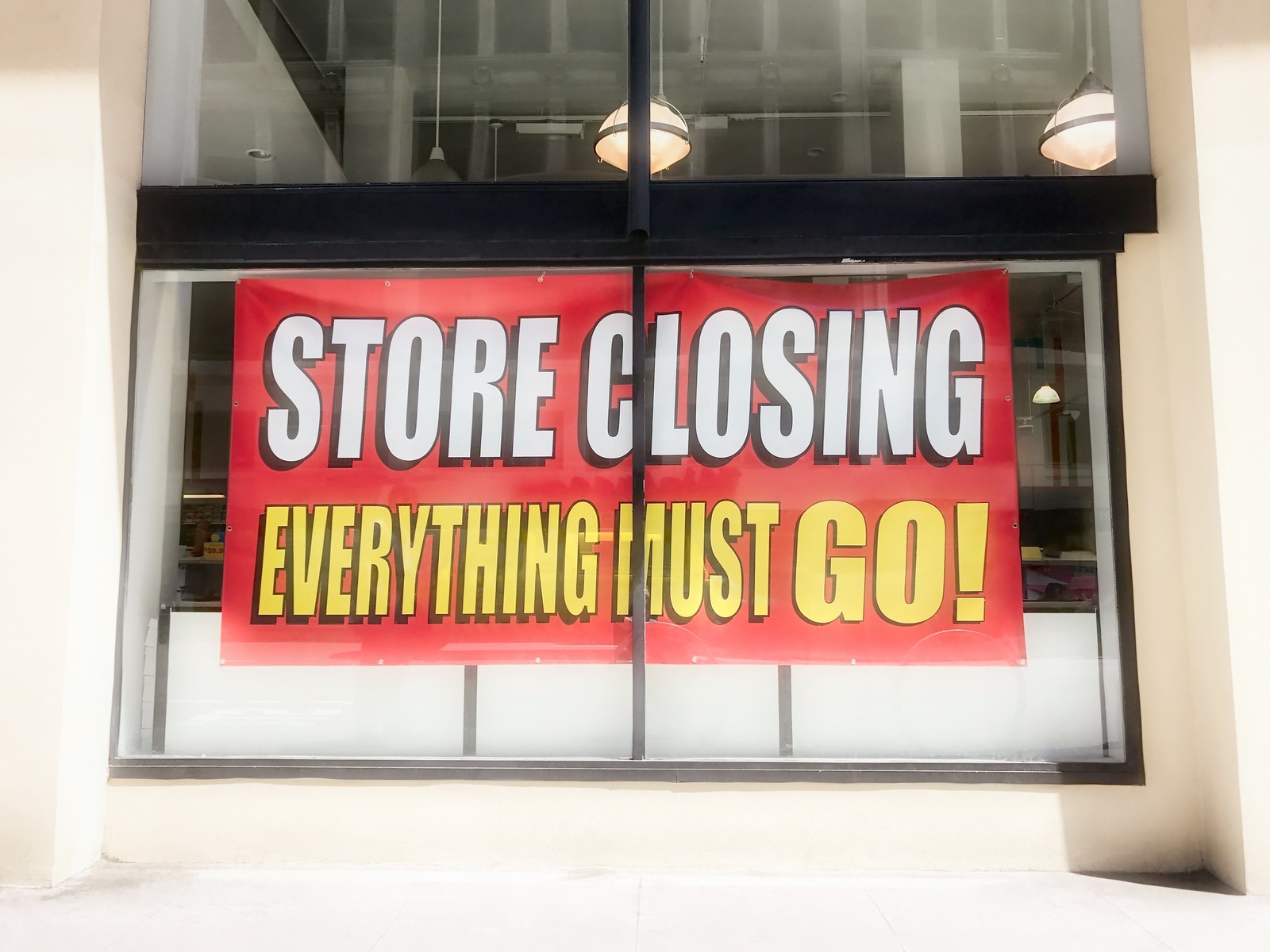This outdoor photograph captures a storefront window adorned with a prominent red sign in bold block letters with drop shadows. The sign announces the store's closure, with the words "STORE CLOSING" in large white letters at the top and "EVERYTHING MUST GO" in bright yellow letters below. Through the window, the interior of the store is partially visible, including a few light fixtures emitting a warm glow. The exterior setting is brightly lit, indicative of a sunny summer day, with the overexposed lighting enhancing the warm atmosphere. The white stucco walls framing the window on both sides and the concrete floor beneath add to the bright and sharp contrast of the scene.